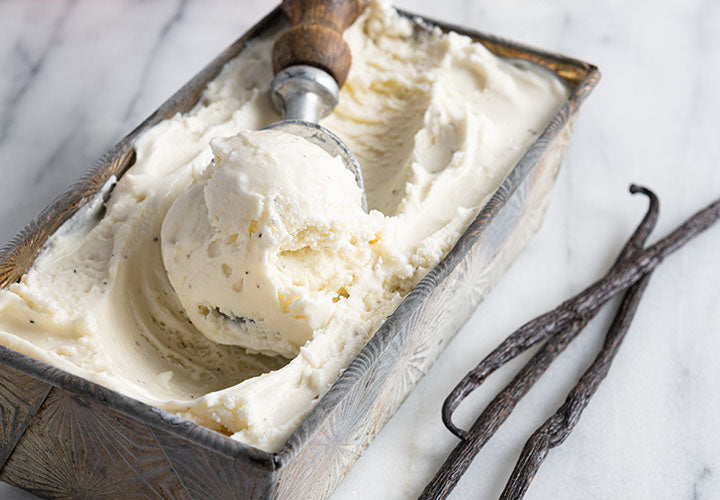The image showcases an intricately carved, vintage wooden box holding a scoop of vanilla bean ice cream. The box features detailed circular and starburst designs, reminiscent of delicate fireworks or sun rays, and exhibits a mix of aged grey and small brown hues, adding to its antique charm. A well-used, vintage ice cream scoop with an old, brown wooden handle is inserted into the ice cream, which displays the characteristic specks of vanilla beans. The entire setting rests on a white and black marble countertop. To the right of the box, three vanilla beans are placed, underscoring the homemade nature of the ice cream. The photograph captures a close-up view, emphasizing the artisanal feel of the scene.